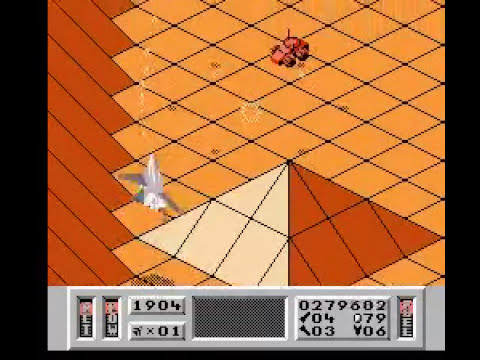The image depicts a vintage video game with a black background. The main visual elements are arranged within the central and right sections of the screen, featuring tanned squares with black lines indicating ground or terrain. A small pyramid composed of lighter tan squares is prominently located in the foreground. On the left-hand side, there's a vertical wall made of long, skinny dark brown rectangles. At the bottom, a rectangular interface possibly displays game information, including the numbers "1904" in black, "Time 01," and other scores. The colors in the image range from black and various shades of brown to white and gray. The overall quality is reminiscent of late 80s or early 90s video games, giving it a nostalgic, retro feel. Notably, a white object resembling an airplane and possibly a tank can be identified within the scene, enhancing the complexity of the game's aesthetic.